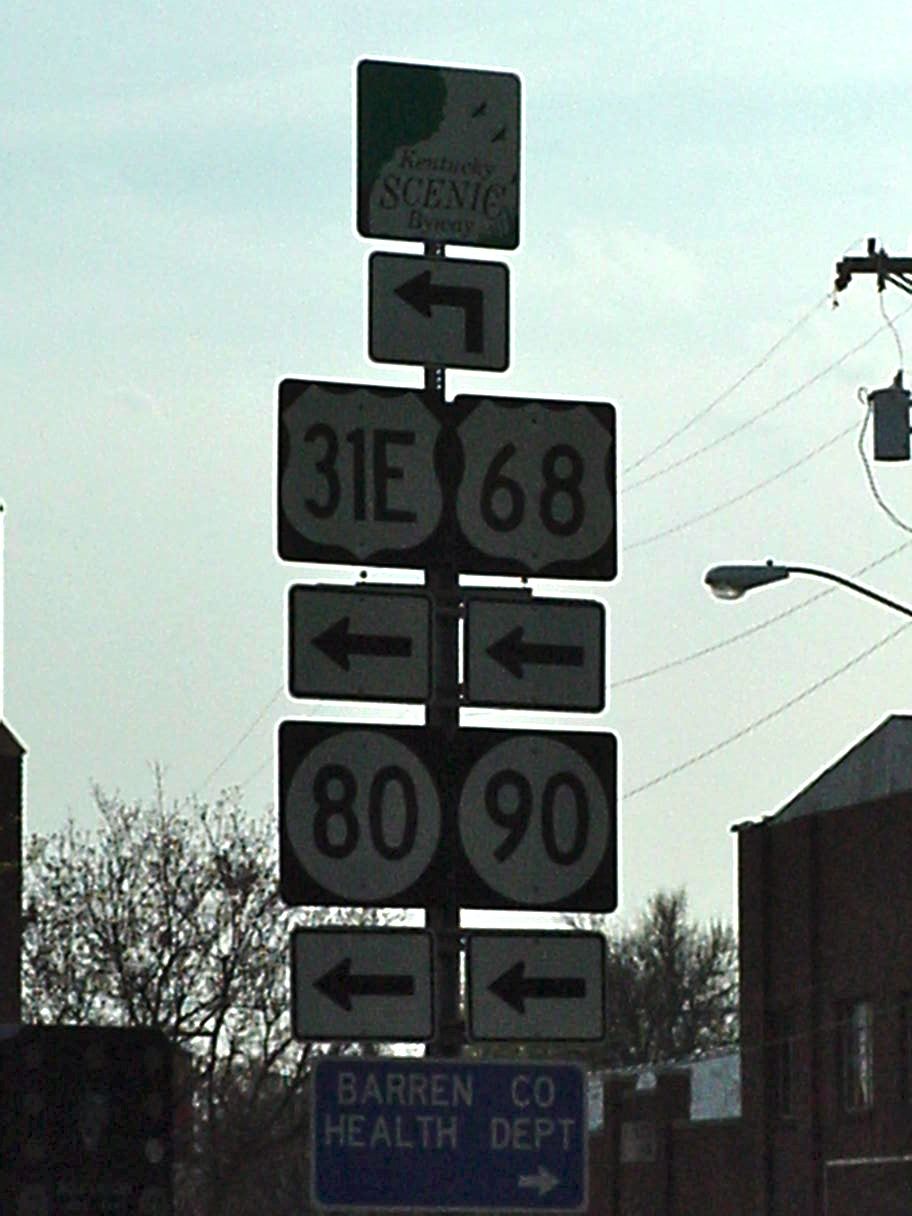This photograph, taken outside during the late afternoon, depicts a series of street signs affixed to a single metal post set against a backdrop of a pale grayish-blue sky. At the top of the post, a white sign featuring three birds and the text "Kentucky Scenic Byway" heralds the start of the markers. Directly beneath it, an arrow points to the left. Following this, a sign with the text "31E68" in dark black writing is displayed. Below it are two smaller signs with left-pointing arrows, succeeded by another sign displaying the numbers "80 90." Two additional left-pointing arrow signs follow this. At the very bottom, a blue sign with white text reads "Barron CO Health Department," accompanied by a right-pointing arrow. On the right side of the image sits a large reddish brick building, while to the left stands a barren tree with only a few remaining leaves, suggesting it may be winter or late autumn. The image is slightly blurry with visible signs of low quality.